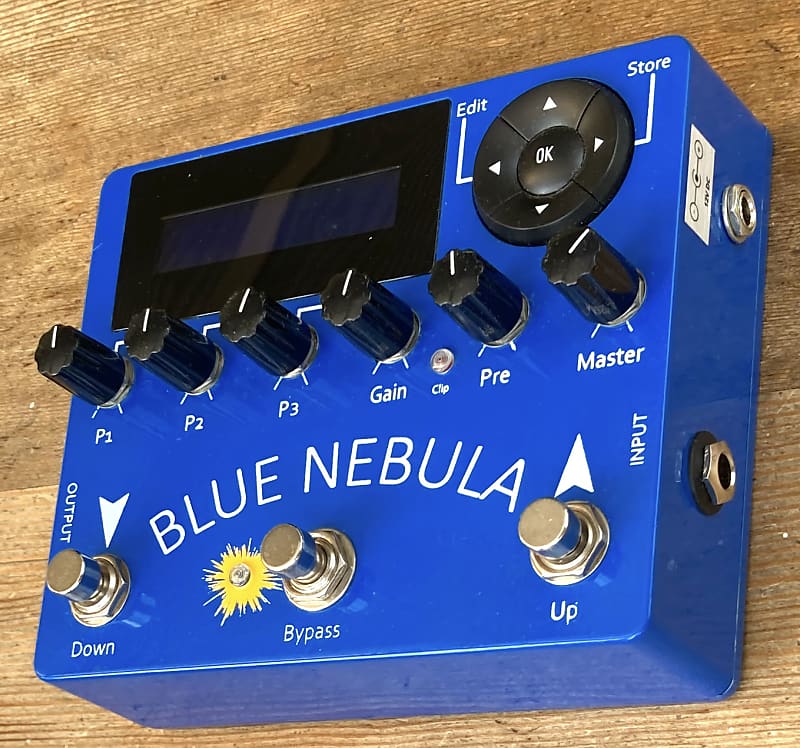The photograph captures a blue metallic audio device with rounded corners, resting on a light brown wooden surface. The device, known as the "Blue Nebula," features a polished and reflective finish. The upper left corner houses a small digital display, while the upper right area is equipped with a control pad consisting of four directional arrows and an OK button, with labels "Edit" and "Store." Below this, in the central part of the device, there are six grooved dark knobs labeled "Master," "Pre," "Gain," "P1," "P2," and "P3." Lower down, the three metallic buttons labeled "Down," "Bypass," and "Up" are arranged horizontally. There are circular holes on the right side for input and output connections. The device's name, "Blue Nebula," is prominently displayed in an arc-shaped text at the lower section.